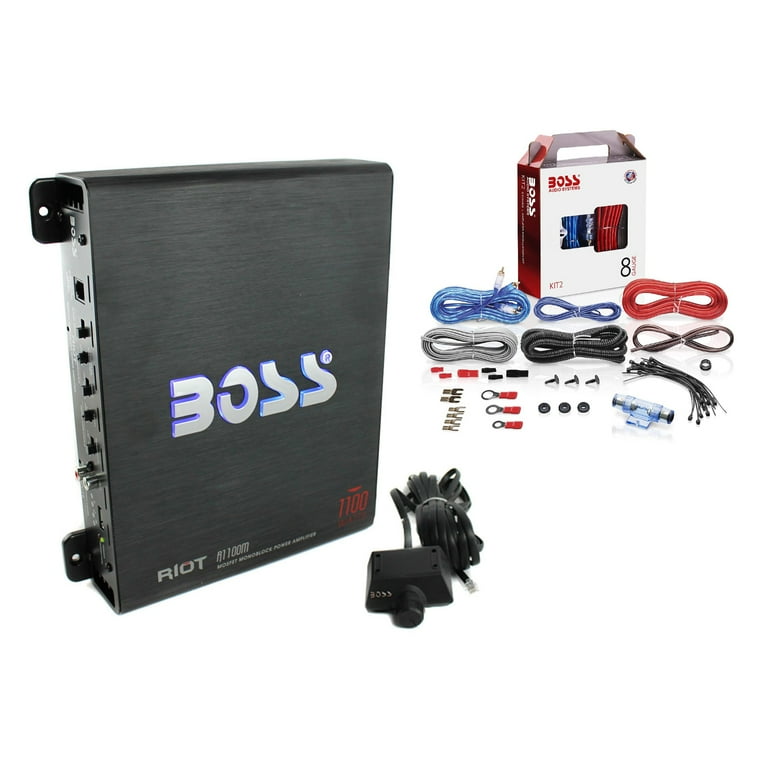The image features a BOSS Riot Power Amplifier, model 1100, prominently displayed on a white background. The large, black metal box, which resembles a computer modem, has white text on the front where the letters "BOSS" are stylized, with the "B" looking like a backward "E" and the "S" missing part of its top curve. Below "BOSS," the word "RIOT" is clearly visible, and the number "1100" is marked in the right corner, though slightly obscured by the angle. This amplifier includes switches and ports on the back, near which an assortment of cords and cables are laid out. 

In front of the amplifier, there is an electrical cord, and to the right, the packaging box the amplifier came in can be seen. This box is white with red detailing and features a handle. Various cables are scattered around the amplifier and its box, including a large blue cable, a small blue cable, a large red cable, a large gray cable, a large black cable, and a small red and black cable. Additionally, the scene includes plastic zip ties and several small metal pieces and gadgets, such as screws and other odds and ends, adding to the technical and cluttered appearance of the setup.